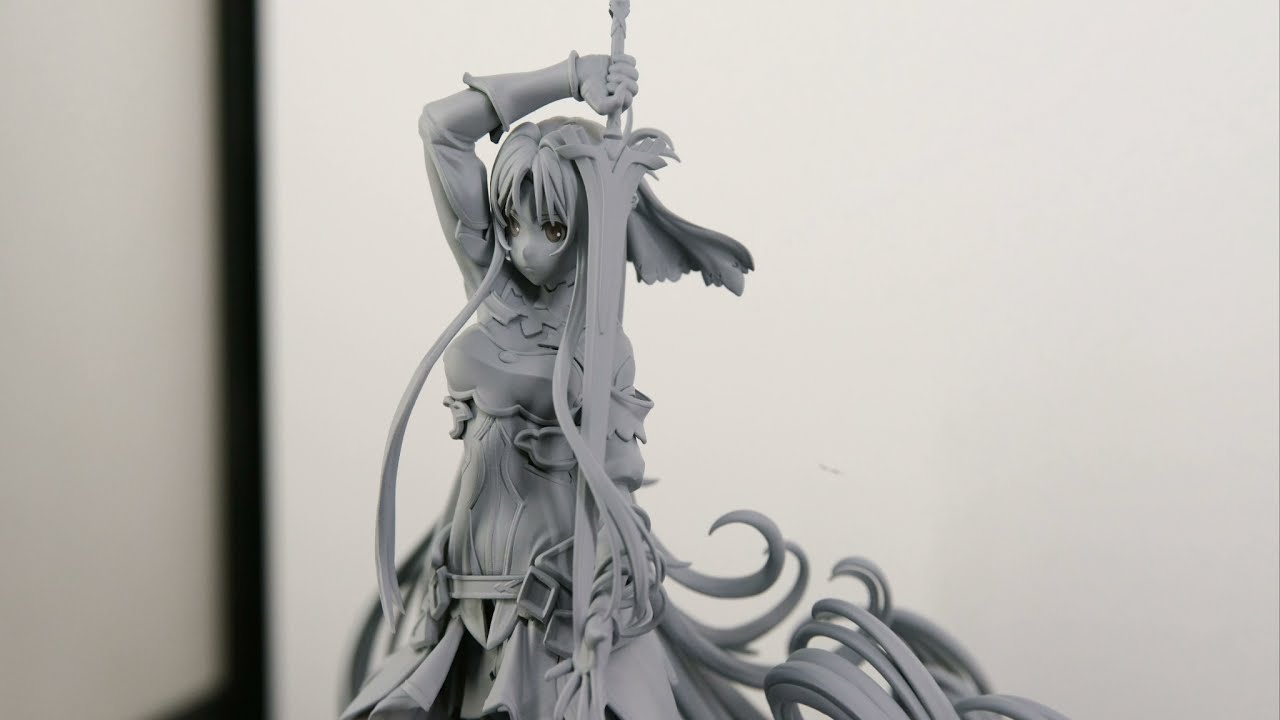In the center of this image, set against an off-white background with a hint of tan on the left and a black crease, stands a highly detailed, gray figurine of an anime girl. The figurine depicts a long-haired female warrior in an aggressive, yet artistically poised stance. She has one arm raised above her head, gripping a large, ornate sword, which she holds pointing downward. Her other hand extends to grasp the tip of the blade, adding to the imposing yet graceful posture. The girl’s detailed costume features flowing robes and intricately designed belts, showcasing the quality of the sculpt, which may suggest it was 3D printed. The figurine, which is centrally placed in the image with an anime-like appearance, includes slightly yellow eyes that contrast with the otherwise monochromatic scheme of whites, blacks, and grays. The background is simple and flat, emphasizing the figurine’s elaborate details and craftsmanship, making it a collectible piece for anime enthusiasts.